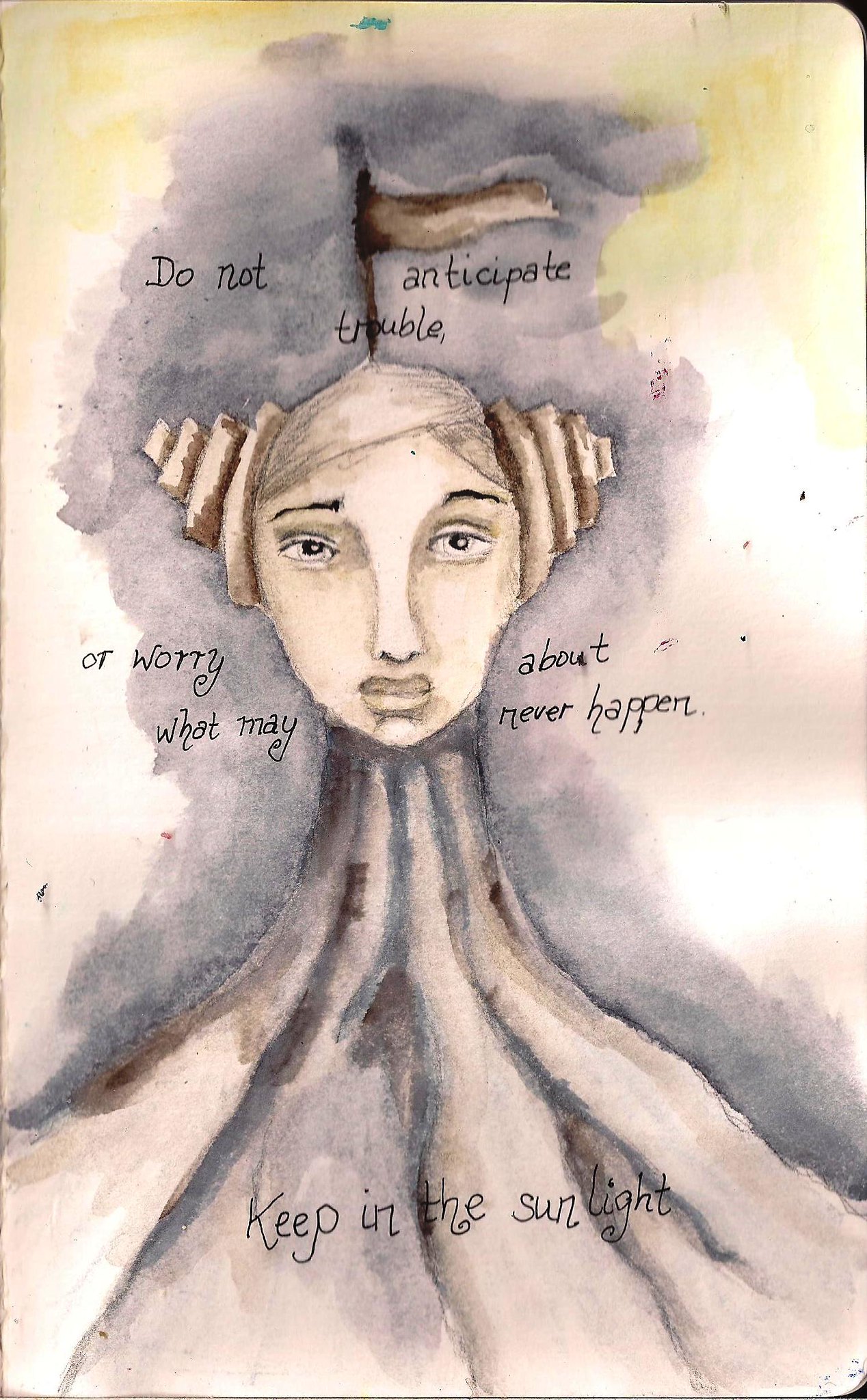The artwork is a watercolor and typography illustration, featuring a purplish-grayish misty background evocative of a smoky volcano. At the center of the painting is the prominent figure of a woman with distinct, elongated facial features, including a long nose, big eyes, and prominent lips. She has short hair with braided headdress-like elements on either side above her ears that resemble cinnamon rolls, adding an otherworldly, almost alien appearance. A beige flag is mounted atop her head. She is dressed in a purple-like outfit and is depicted with a slightly upward, straight-ahead gaze and a sad expression. Overlaying the image in black script, fragmented text reads, "Do Not Anticipate Trouble" across the top of her head. The text continues, "Or Worry, What May, About, Never Happen," around her face, and finishes with "Keep in the Sunlight" written across her chest. This detailed composition blends watercolor illustration with graphic design typography to capture a surreal and contemplative scene.